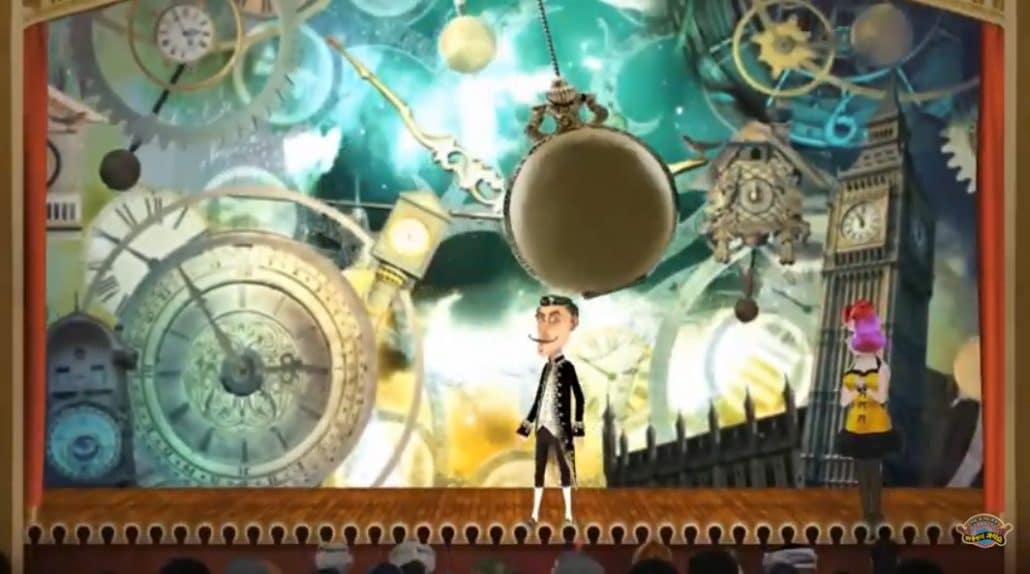This intricate, colorful artist's sketch portrays a vibrant, cartoonish stage set brimming with a diverse array of clocks. The stage is framed by rich red curtains and illuminated by footlights. At the center stage, a dapper white man with a pencil-thin mustache, dark hair, and a formal long-tail black coat, black breeches, and white stockings stands poised. To his right, a striking female figure with elaborate purple and red hair dons a knee-length, low-cut yellow dress with black trim and black stockings. 

Behind them, the background bursts with clock-themed motifs, including the iconic Big Ben clock tower, ornate wall clocks, cuckoo clocks, and street corner clocks all interspersed with pocket watches, pendulums, and gears. In the lower left corner, a unique double cuckoo clock with animated figures adds whimsical charm. Clocks in silhouette and in distant forms create depth, while assorted pendulums and springs in the upper right corner contribute to the mechanical maze. The overall scene is enveloped in a reddish-brown mat and a dark brown wood-like frame, adding a vintage touch to this dynamic tableau.